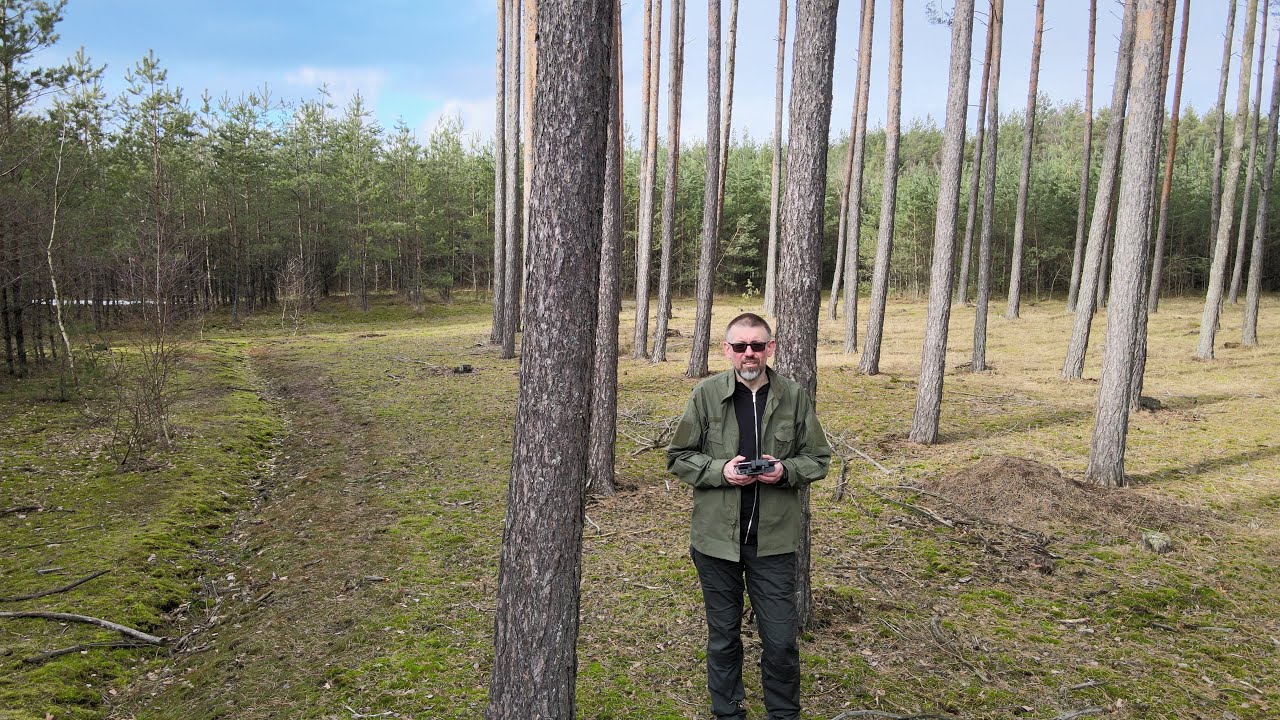In the center of the image, taken at a grown man's head height, a man stands facing the camera. He is wearing dark sunglasses and a green jacket over a possible black sweatshirt. His short, gray-flecked hair and beard suggest he is probably in his 40s or 50s. He's holding a device that could be a controller for a drone or a camera. The man stands slightly off-center to the right of the frame, beside a tree trunk, amidst a grove of tall pine trees with bare trunks and no visible branches. To the left of the man, there is a lightly treaded path. The background features a dense array of trees with leaves, contrasting with the leafless pines in the foreground. The blue sky peeks through the tops of these trees, indicating it's daytime. The ground in the foreground is cleared with patches of green grass. The overall setting is a serene, forested nature area.